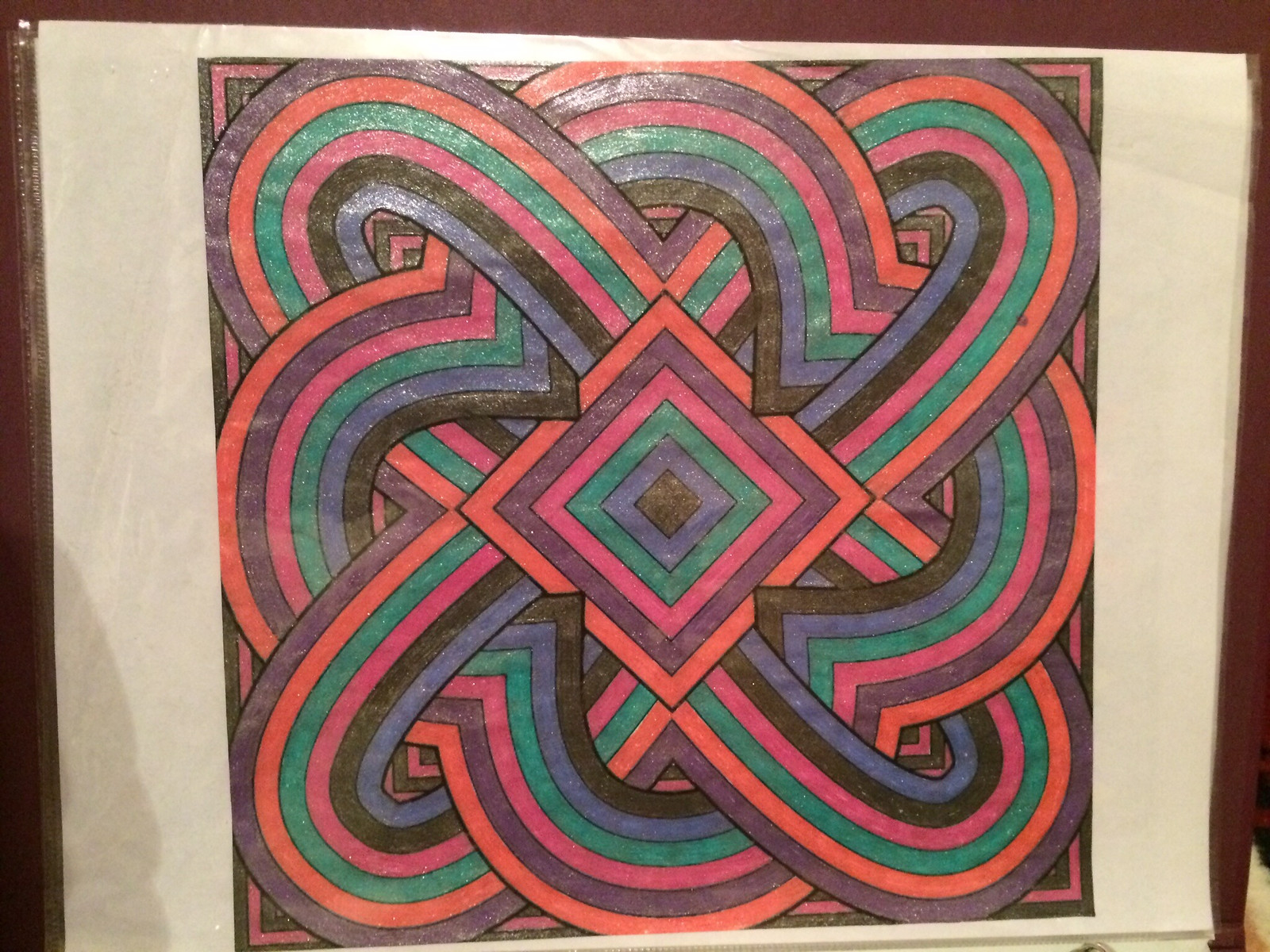This vibrant artwork features a central diamond-shaped figure, created by rotating a square. The diamond contains intricate, layered designs that evoke a sense of depth and dimensionality. Radiating from this central element, sweeping lines form large U-shaped patterns that flow both into and out of the diamond, creating a dynamic movement throughout the piece. The composition is rich with an array of colors, including blues, purples, pinks, reds, and oranges, giving it a lively and captivating aesthetic. The texture suggests that the art was crafted using crayons or pastels, adding a tactile quality to the visual experience.